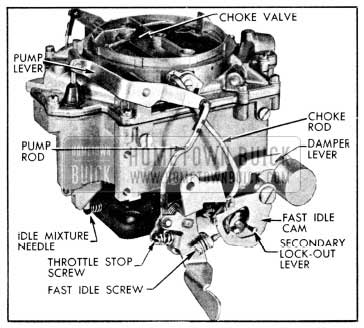This is a highly detailed and hyper-realistic black and white schematic, resembling a hand-drawn or pencil-sketched illustration, of a mechanical part likely related to a vehicle, given the watermark "Hometown Buick". The schematic meticulously labels various components using arrows pointing to specific parts. Notable elements include the choke valve, pump lever, pump rod, idle mixture needle, throttle stop screw, fast idle screw, secondary lockout lever, fast idle cam, damper lever, and choke rod. The intricate depiction showcases a square mechanism with a circular top featuring multiple moving parts such as levers and springs, all contributing to a comprehensive understanding of the machinery’s inner workings.